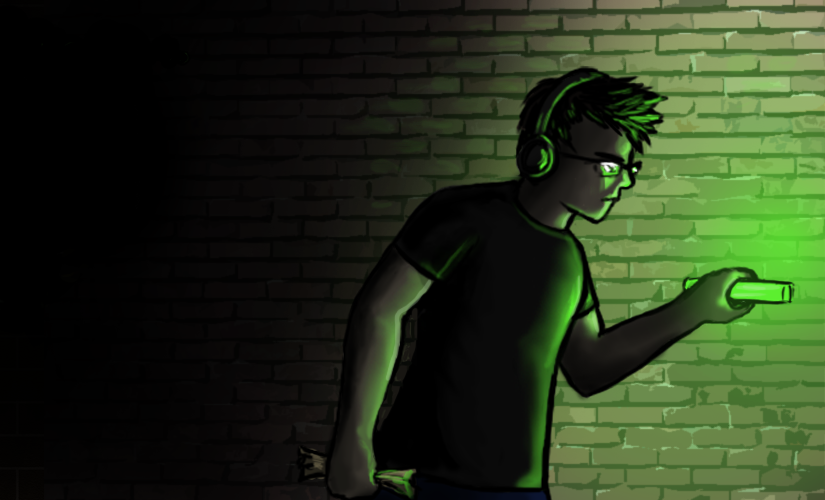The image depicts a digitally drawn cartoon of a young man with spiky black hair, illuminated by a green glow stick in his left hand that casts a neon green light on his hair strands and surroundings. The young man is wearing green glasses and headphones, along with a black short-sleeved t-shirt. In his right hand, he holds a newspaper, and his serious, focused expression suggests he is investigating something. He is positioned against a red brick wall, which transitions into a fade of darkness on the left side of the image, enhancing the sense of him walking through a dimly lit environment. The brick wall features a blend of green and black, adding to the eerie, investigative atmosphere of the setting.